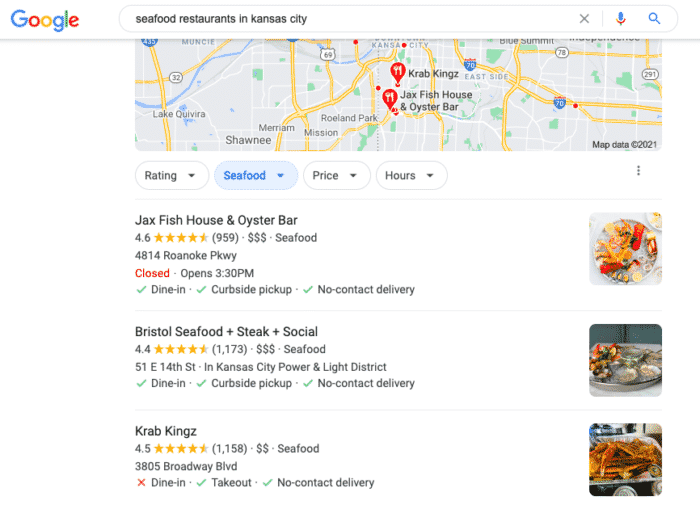**Detailed Caption for Google Search Screenshot:**

The image is a screen capture of a Google search with the distinctive blue, red, golden, and green Google logo. The interface appears to feature a specialized theme with subtle dividing lines. In the search box, "seafood restaurants in Kansas City" is entered in black text. Adjacent to the text box are interactive symbols: a gray 'X' to clear the search, a multicolored microphone for voice input, and a blue magnifying glass icon to initiate the search.

Below the search bar, there's a Google Maps section with a 2021 copyright notice at the bottom. The map displays two red location pins with white knife and fork icons. The first pin marks "Crab Kings," and the second marks "Jack's Fish House and Oyster Bar."

Scrolling further, options to sort results by rating, type of seafood, price, and hours of operation are presented. These filters, highlighted in blue, can be expanded using pull-down arrows, and three gray dots indicating additional settings are aligned to the side.

The first search result lists "Jack's Fish House and Oyster Bar," rated 4.6 stars with 959 reviews. It features three dollar signs, indicating a higher price range, and identifies the location as 4814 Roanoke Parkway (PKWY). The status notes it is currently closed and will open at 3:30 PM. The restaurant offers dine-in, curbside pickup, and no-contact delivery, each verified with green check marks. The result includes a gold and red hued food image.

The next result is "Bristol Seafood + Steak + Social," with a 4.4 star rating from 1173 reviews. It also has three dollar signs, suggesting similar pricing, and is located at 51 East 14th Street, Kansas City Power and Light District. The same green check marks confirm availability of dine-in, curbside pickup, and no-contact delivery options. A picture showing oysters accompanies this entry.

The final listing is "Crab Kings," boasting a 4.5 star rating from 1158 reviews with two dollar signs, indicating a more moderate price range. Situated at 3805 Broadway Boulevard, this establishment offers takeout and no-contact delivery, each validated with green check marks. Notably, dine-in service is marked with a red 'X', signaling unavailability. An image of a fish dish in a styrofoam container is displayed alongside this listing.